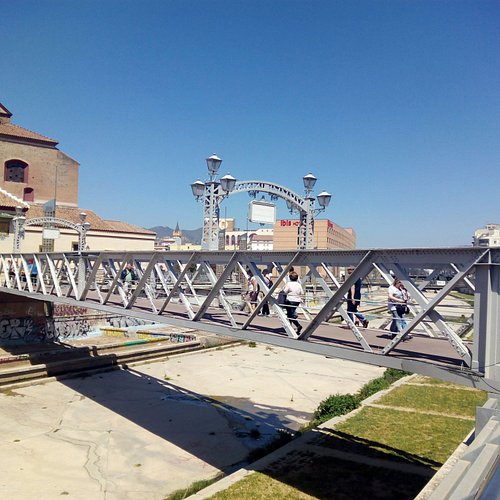The photograph captures a detailed and vibrant scene of a pedestrian bridge on a clear, sunny day. The steel bridge, painted grayish-white, arches over a dry canal with a cement bottom and sides, interspersed with patches of greenery. The bridge features crisscrossing girders and three cables on each side, with the tall railings towering above the heads of pedestrians who are seen walking back and forth. Shadows of the bridge cast intricate patterns over the canal below. On the right side, a cement retaining wall is bordered by manicured grass and sidewalks leading up to it.

In the background, a multi-story brick building, likely two or three stories tall, is visible on the left. Further to the left rises an archway with lanterns, made from matching steel. This bridge appears to connect to buildings that could potentially be office spaces or a hotel, suggested by barely visible red text on one of the beige-walled structures. The scene is serene, with expansive blue skies and rolling hills in the distance punctuated by the silhouette of a church steeple or tower. Large light fixtures stand out in the distance, adding to the urban but tranquil ambiance of the area.